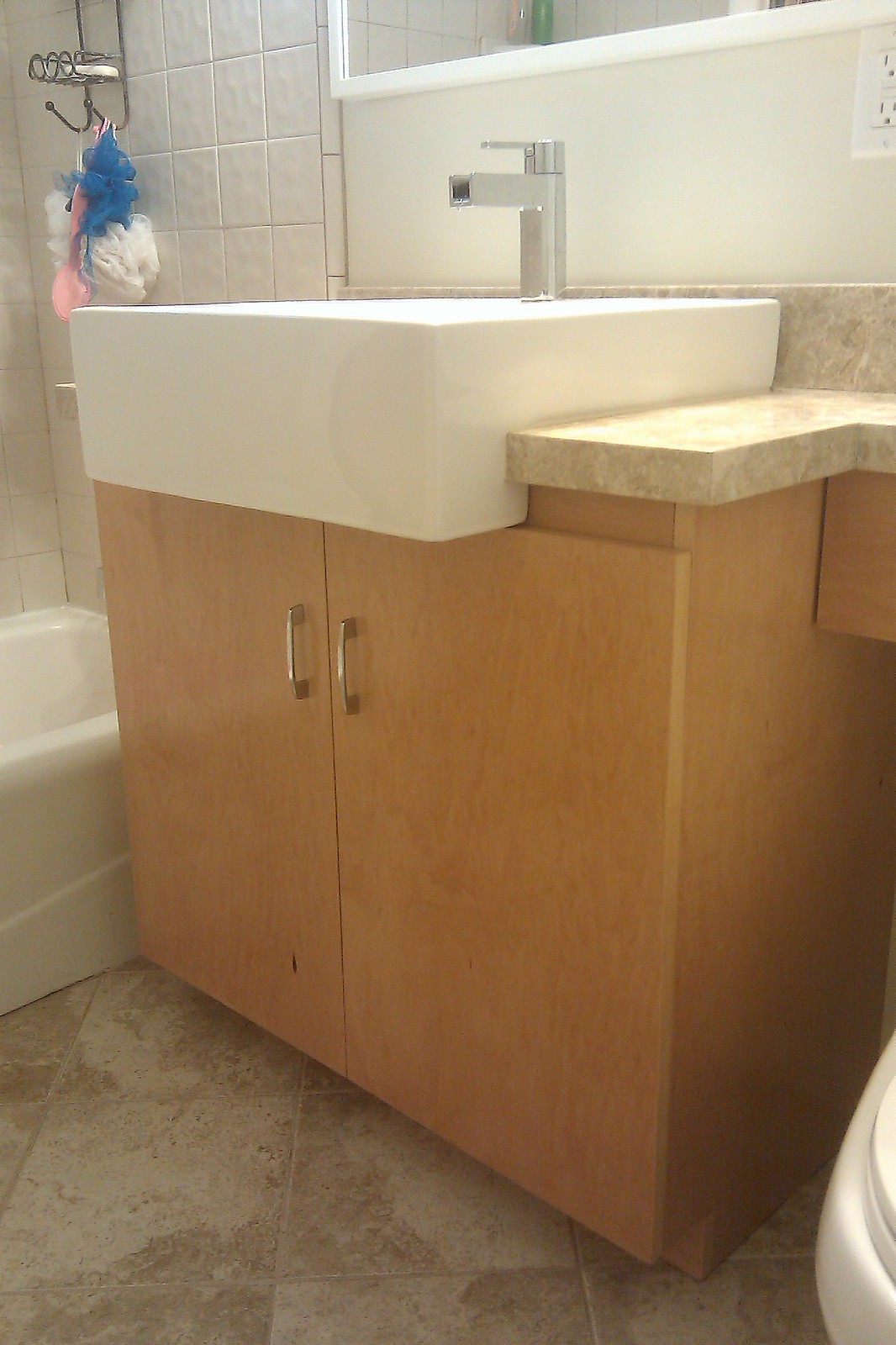This photo captures a serene and modern bathroom centered around a stylish sink. Taken from a low angle, the image showcases a light brown wooden cupboard beneath a large, rectangular white stone sink, positioned at the focal point. The sink rests upon a sleek, one-and-a-half-inch thick tan marble countertop, accentuating the luxurious feel. The bathroom floor features tan stone tiles with varied textures, adding depth and interest to the space. A distinctive rectangular faucet, with an exposed design allowing the water to be seen flowing, complements the sink's modern aesthetic. To the left of the sink, partially visible, is a bathtub or shower area adorned with hanging loofahs on a convenient rack. Adjacent to the sink on the right is a toilet, completing the essential elements of this tastefully designed bathroom.